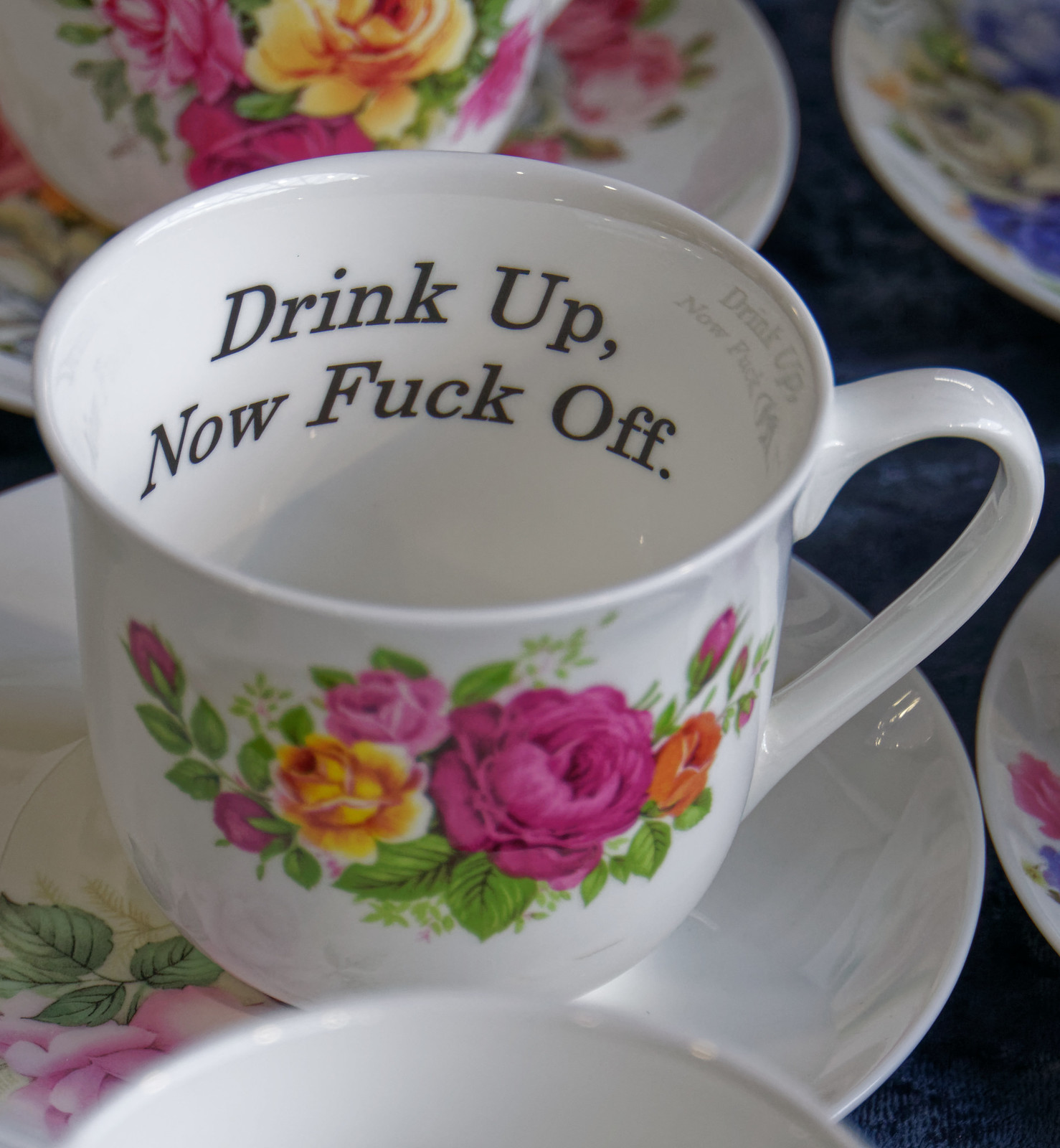This detailed image showcases a central white porcelain teacup adorned with a vibrant floral pattern featuring a pinkish-red carnation, a yellow flower, and what appears to be an orange tulip, amongst smaller magenta flowers and lush green leaves. The teacup rests on a matching saucer, which also carries a floral motif, including green leaves and a pink flower. Inside the teacup, an unexpected and bold message in italicized black text reads, "Drink up, now fuck off." This central teacup is surrounded by other similar teacups and saucers that are partially visible, slightly blurred, and out of focus against the backdrop of a dark navy blue tablecloth, emphasizing the central composition's elegant yet audacious contradiction.